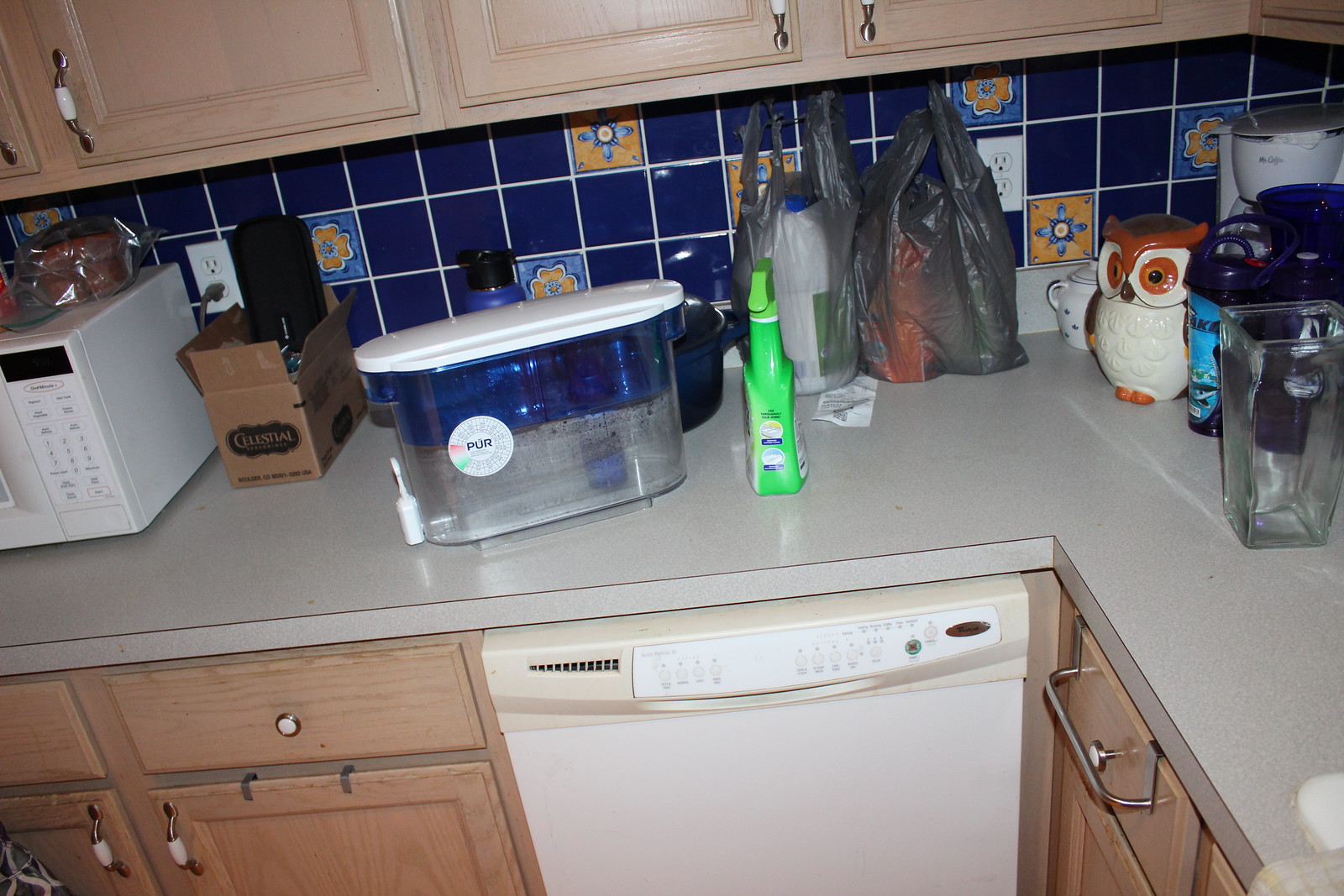The image depicts the right corner of a kitchen featuring an L-shaped countertop painted white with a glossy finish, likely made of wood. The light wooden cabinets with gold handles, accented with a white piece in the center, add a touch of elegance. To the left, part of a white microwave is visible, topped with packaged bread and a small cardboard box beside it. A long, oval-shaped water purifier stands next to the microwave, with a green bottle cleaner facing the wall behind it. Two plastic bags containing more cleaning supplies are tucked behind the purifier. In the corner of the countertop arrangement, there is an owl sculpture, several water bottles, and a clear vase. Behind these items, the top of a white coffee maker is slightly visible. Below the green bottle cleaner is a white dishwasher. The kitchen backsplash consists of blue tiles interspersed with blue and orange tiles featuring floral designs.